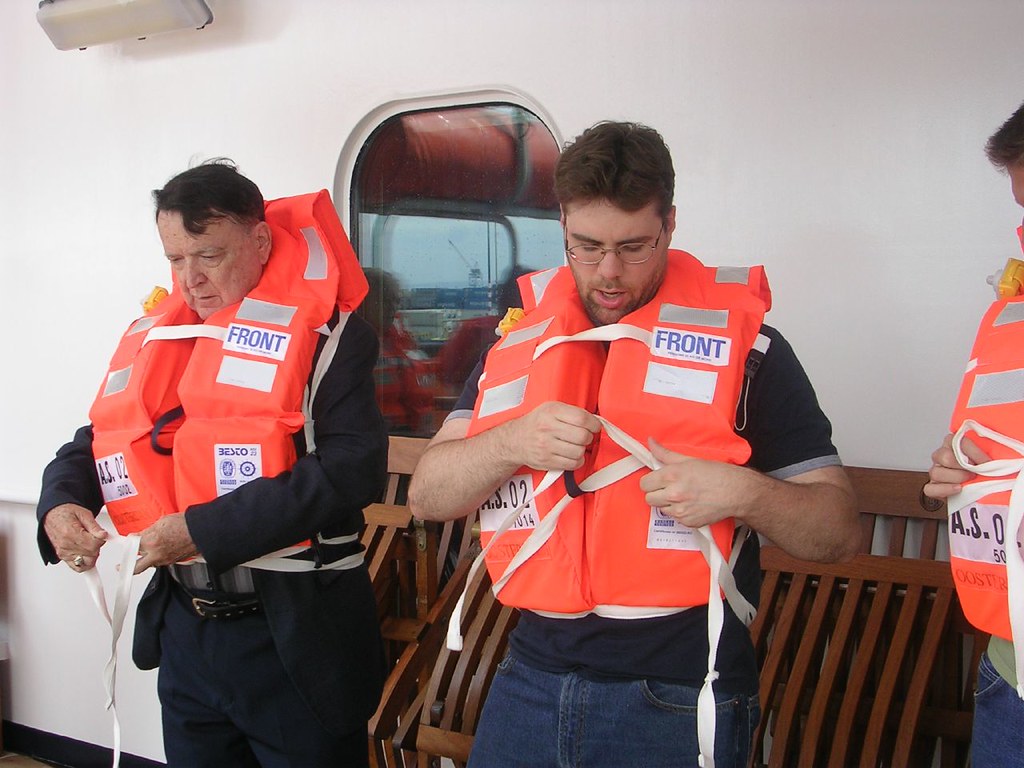In this close-up photograph, three men are in the process of learning to put on bright orange life vests on what appears to be a white boat docked in a marina. The backdrop behind them is a white metal wall, and a rounded window reflects another boat and possibly an antenna or crane, indicating they are still docked. The focal points are the men centered in the image. The man on the left is elderly with sparse black hair, fair complexion, and wearing a black suit with a silver buckle tie, black belt, and black pants. He is adjusting his life vest, which has white straps and patches labeling 'Front' in blue text. He also wears a ring on his right hand ring finger. 

To his left, a younger man with brown hair and a beard, dressed in a black t-shirt and navy blue jeans, is also securing his life vest while wearing glasses. His vest, similar to the elderly man's, features white ties and multiple reflective silver rectangles, with patches labeled 'Front' and 'ASO2.'

The third man to the far right is partially cropped out of the frame but is dressed in a green shirt and jeans. Together, the three are focused on correctly fastening their life vests, with the two visible men diligently working on their task amidst the safety demonstration. Brown wooden benches, folded up, are also visible along the sides, suggesting the deck area of the boat.